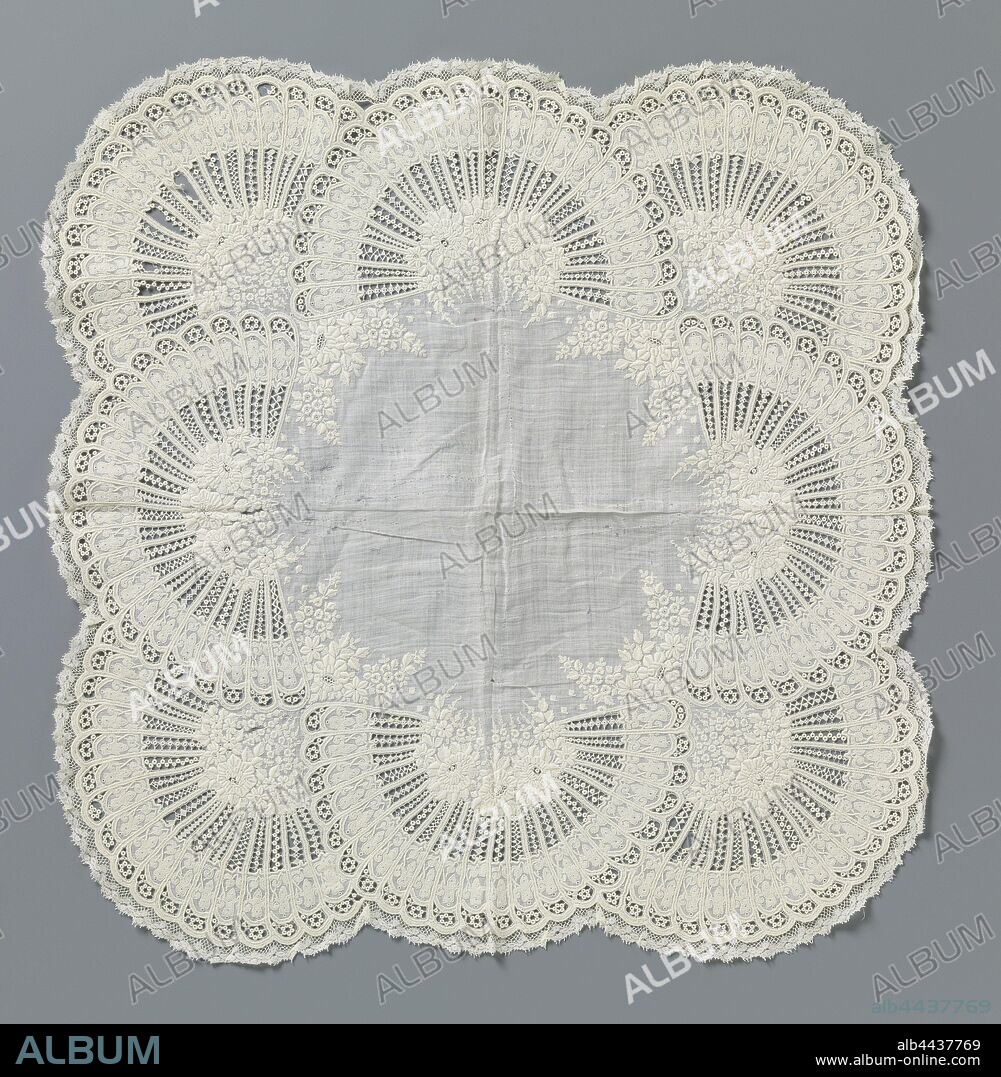The image is a photograph featuring an array of nine circular white doilies, which could be either cloth or paper, arranged in a three-by-three formation with slight overlaps on a gray background. The doilies exhibit a detailed lace or crochet pattern. Superimposed across the entire image is the word "album," which is slightly difficult to read due to its white color blending with the doilies. At the bottom of the image, a black horizontal banner contains additional text: on the left side, it says "album," and on the right, it features a serial number, "ALB4437769," followed by the website "www.album-online.com." The photograph appears to be a web page snapshot or an advertisement for the brand "album," highlighting decorative lace patterns on a minimalistic gray and black design.